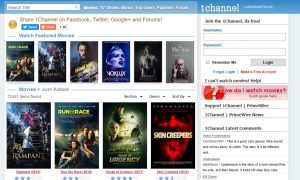The image displays a channel website interface which appears to either host movies or book covers. The content is highly condensed, making specific details difficult to discern. The website features a clean white backdrop with blue accents. At the top, there is a blue-bordered area, and on the left-hand side, there is a search bar accompanied by six menu options written in white text.

The layout is divided into two primary sections. The right-hand side contains a section labeled "One Channel," followed by text in black that isn't fully legible. Below this are fields for entering a username and password, along with a checkbox for "Remember me" and a "Login" button. Directly beneath the login section, there's a blue hyperlink labeled "Forgot login?" and a red text mentioning the word "account," followed by some unreadable black text that includes the word "help." An advertisement is positioned just below this area, and further unidentifiable items are listed beneath the ad.

On the left side, there are ten images arranged in two rows. The first row consists of six smaller images while the second row features four larger images. One image appears to be titled "Sign Creepers," hinting at a scary movie, while another seems to be labeled "Urgency" with additional text reading "Run Race." The bottom row includes a star rating system, indicating user reviews for the visual content.